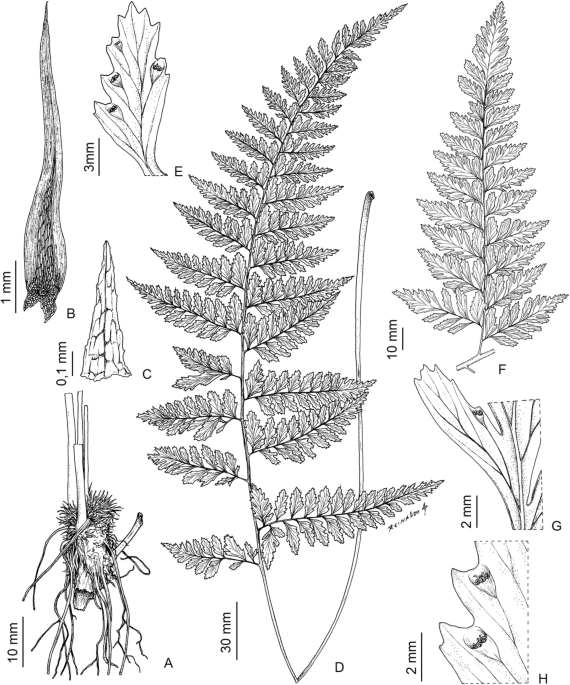This black-and-white print appears to be an illustration from a nature book. It meticulously details various parts of plants, including ferns, leaves, stems, and seeds. The central focus of the page is a tall, tapering fern stem that has fronds extending to the right and left, labeled with a capital D at the bottom, and 30MM to the left. Surrounding this central fern, the illustration includes a series of labeled plant parts and measurements. To the lower left, labeled A, is a clumpy root structure with a few visible roots, marked with 10MM. Above this, the letter B points to a seed or spindly leaf, wider at the bottom and thinning towards the top, alongside a 1MM label. Adjacent to B, the letter C denotes a triangular plant piece with a central black line and ridged edges, while above this, E marks a tall, thin leaf showing seeds along its veins, labeled 3MM. On the right side, F denotes another fern-like plant part, with 10MM. Below this, G represents a half-section of a leaf, revealing its stem and veins, marked with 2MM. At the bottom right corner, an even larger leaf section marked with H displays veins and seeds, labeled 2MM. Each plant part is intricately detailed, creating a comprehensive botanical study.